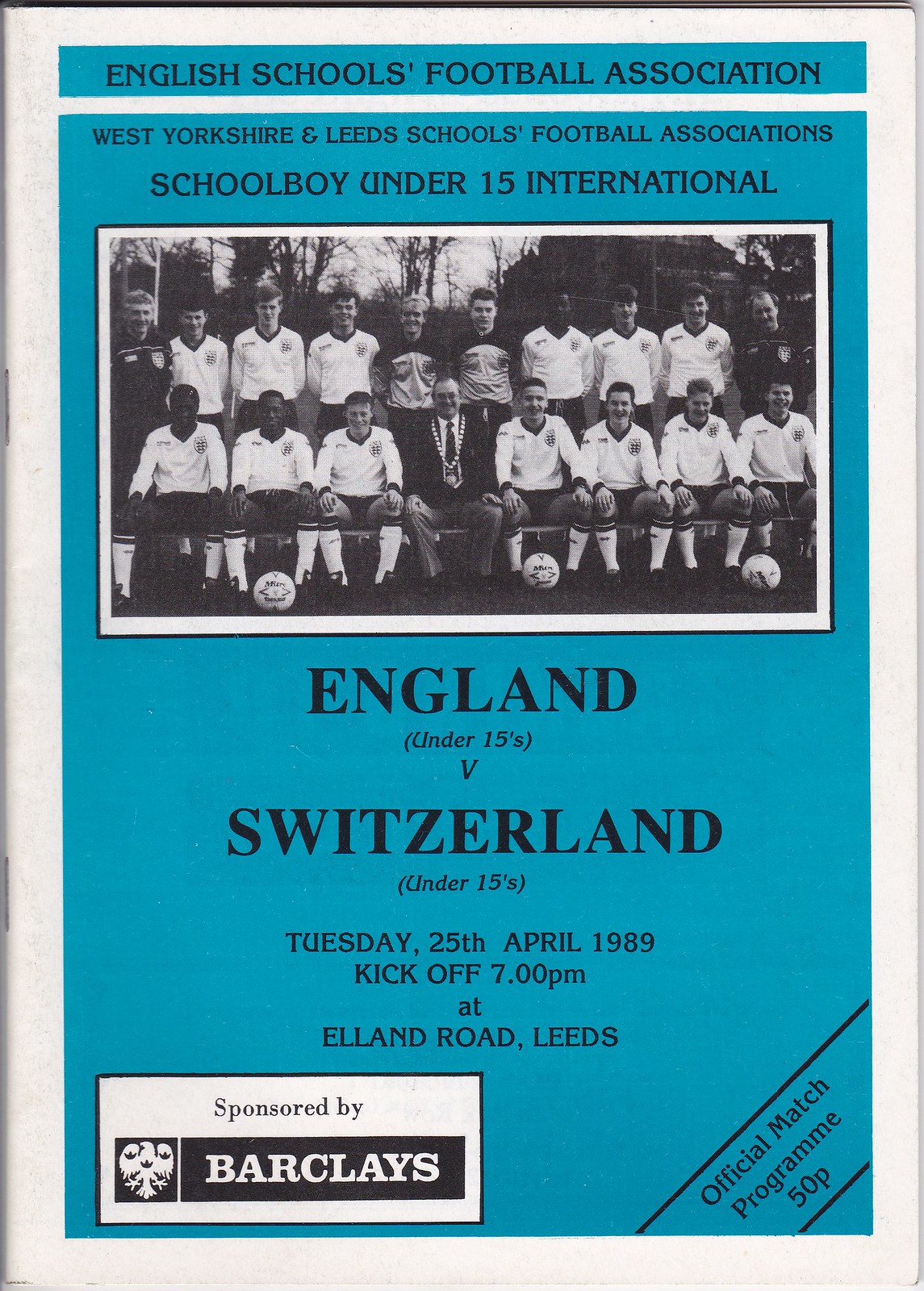This image showcases the front page of an official match program from the 1980s for an Under-15 international football match between England and Switzerland. The page predominantly features a large blue background with a white border on all sides. At the very top, there's a thin blue strip with "English Schools Football Association" written in black text. Below this strip, the program highlights that it is organized by the West Yorkshire and Leeds Schools Football Association.

Central to the design is a black-and-white photograph of a football team, with the front row sitting, the coach in the middle, and the back row standing, all with soccer balls lined up in front of the seated players. Above the image, in black text, it reads "Schoolboy Under 15 International." Below the image, large black letters announce the match: "England v Switzerland." Following this, more text details the date (Tuesday, 25 April 1989), the kickoff time (7 p.m.), and the location (Elland Road, Leeds).

In the bottom left corner is a white triangle with the words "sponsored by" and "Barclays" in large white letters inside a black box. Additionally, the bottom right corner features angled black text between two lines, stating "Official Match Program 50-P."